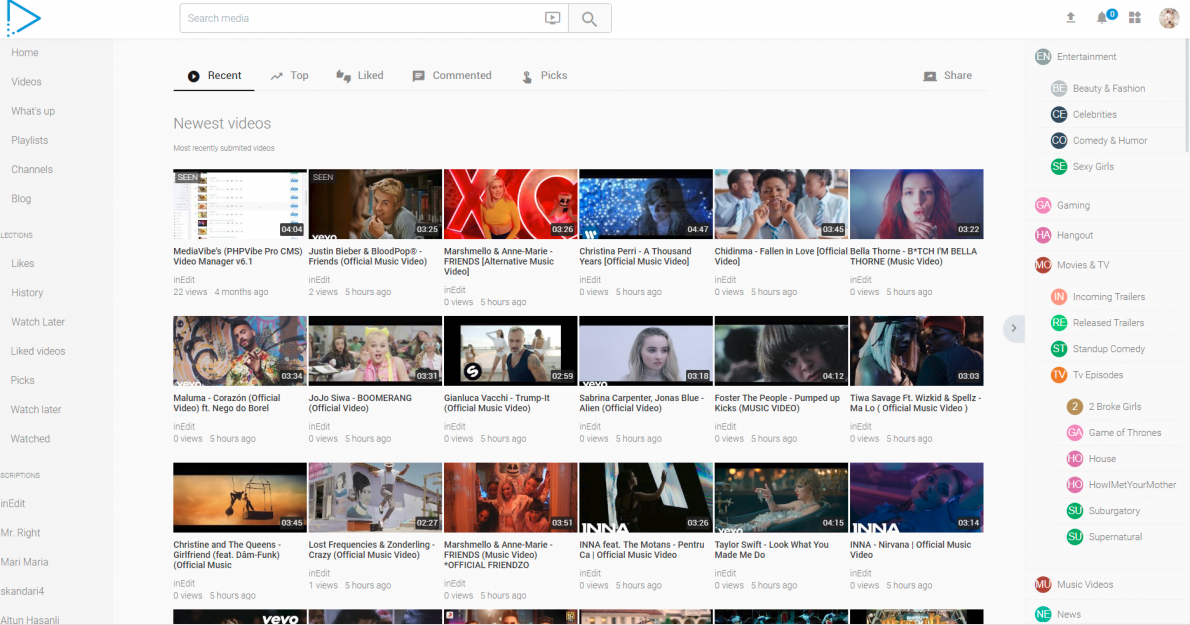The image depicts a webpage resembling YouTube with a predominantly white background. On the far left, there is a vertically oriented drop-down menu. The menu items include a blue arrow pointing to the right, followed by text links that read "Home," "Videos," "Playlists," "Channels," "Blog," and an unreadable item. Further down, it lists "Likes," "History," "Watch Later," and "Watched." At the bottom, options like "Edit" and several unreadable items are present.

In the middle portion of the page, a search bar is located at the top. Below it, there are five tabs labeled "Recent," "Top," "Liked," "Commented," and "Pictures," allowing users to filter content. To the right of these tabs, there's a share button. Under these elements, the section titled "Newest Videos" is visible, displaying three complete rows and a partial fourth row, with six video thumbnails per row.

On the far right, a set of icons is present at the top, although they are indiscernible. Beneath these icons, the word "Entertainment" is followed by a list of subcategories, arranged vertically along the entire length of the page.